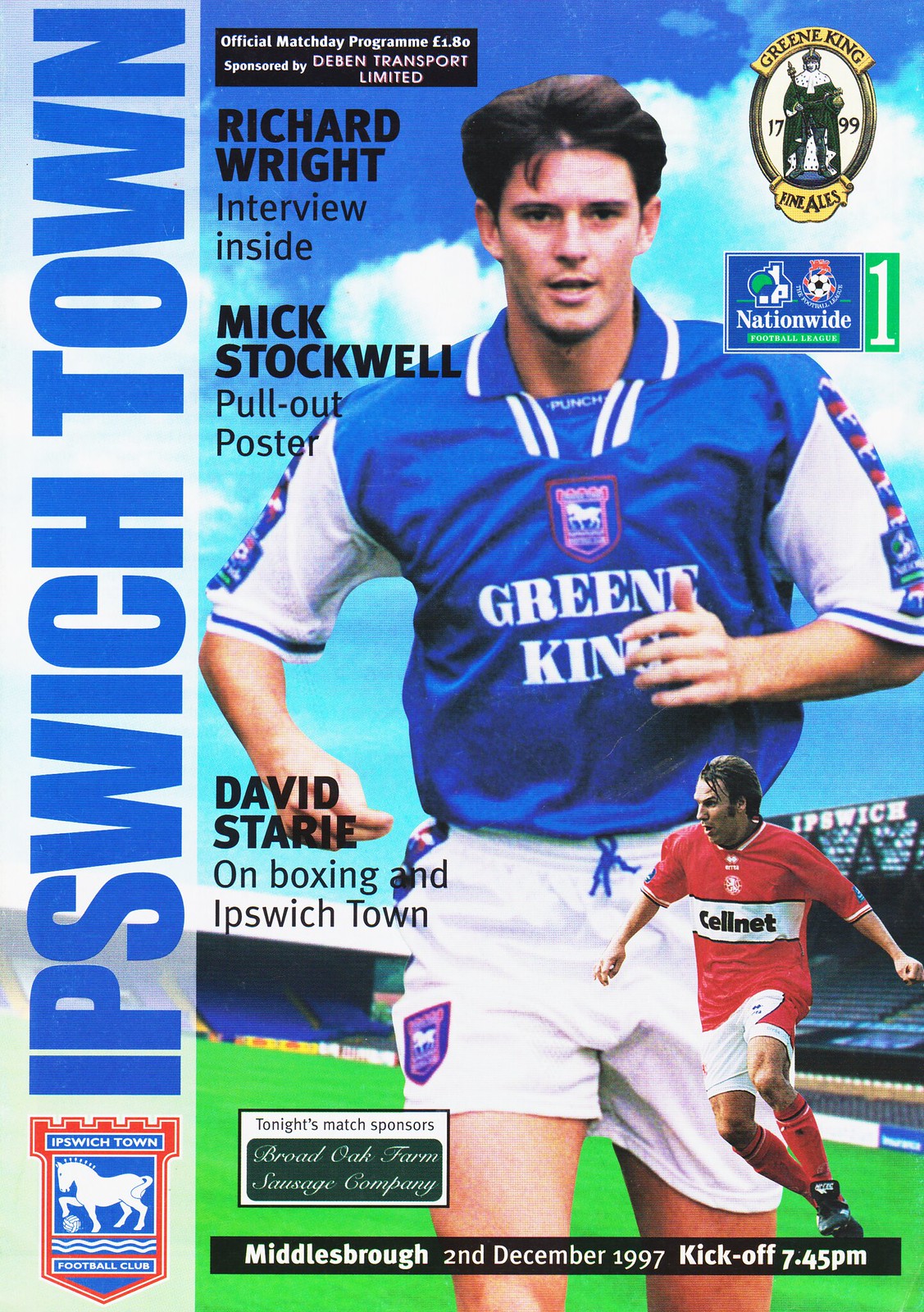The image is a detailed magazine cover featuring promotional content for the sports team Ipswich Town. Running diagonally along the left side in large blue letters is "IPSWICH TOWN," complemented by an emblem featuring a horse in the bottom left corner. The central and right sections of the cover showcase a dynamic action shot of a soccer player with short black hair running forward. He is dressed in a blue and white jersey with the text "Greene King" partially visible on the chest, accompanied by white shorts with team emblems on the sides. 

Superimposed in a smaller inset near his left leg, another soccer player in a red and white jersey is caught mid-run as if about to kick a ball. This inset player wears red socks and white shorts. The background faintly displays a stadium scene with visible green field and blue sky.

The magazine contains several highlighted features: 
- A "Richard Wright interview inside," prominently noted in a black box with white writing near the upper left beside the main player's head.
- A "Mick Stockwell pull-out poster.”
- An article on "David Stary on boxing in Ipswich Town."

At the bottom of the cover, in a black rectangular strip with white writing, the text indicates an upcoming match: "Middlesbrough, 2nd February 1997, kickoff 7:45 p.m."